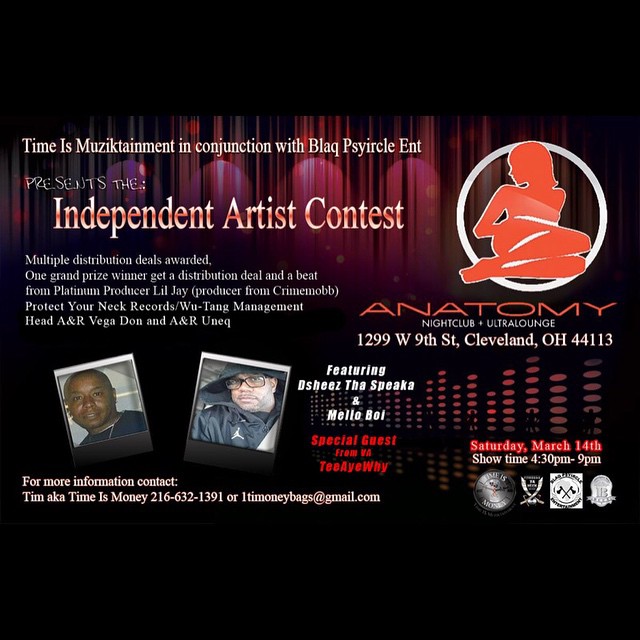The image is an advertisement for an independent artist contest against a black background with red and purple stage curtains. At the top, it reads, "Time Is Music Attainment in conjunction with Black Cyclical Entertainment presents the Independent Artist Contest." Multiple distribution deals will be awarded, and one grand prize winner will receive a distribution deal and a beat from platinum producer Little J of Crime Mob, in association with Protect Your Neck Records and Wu-Tang Management, with Head A&R Vega Dunn and A&R UNEC.

On the right side of the image is a logo depicting a woman seated seductively, looking to her right, encircled in red and white. Below this logo, it says, "Anatomy Nightclub Ultra Lounge, 1299 West 9th Street, Cleveland, Ohio, 44113." The advertisement features special guests Oshie's, The Speakah, and Mellow Boy, with a special guest appearance from TIY. 

In the bottom left corner, there is a photograph of two African American men with contact information, stating: "For more information, contact: Time Is Money, 216-632-1391, or onetimemoneybags@gmail.com." The bottom right corner of the image includes additional logos and specifies the event date and time: "Saturday, March 14th, from 4:30 PM to 9 PM."